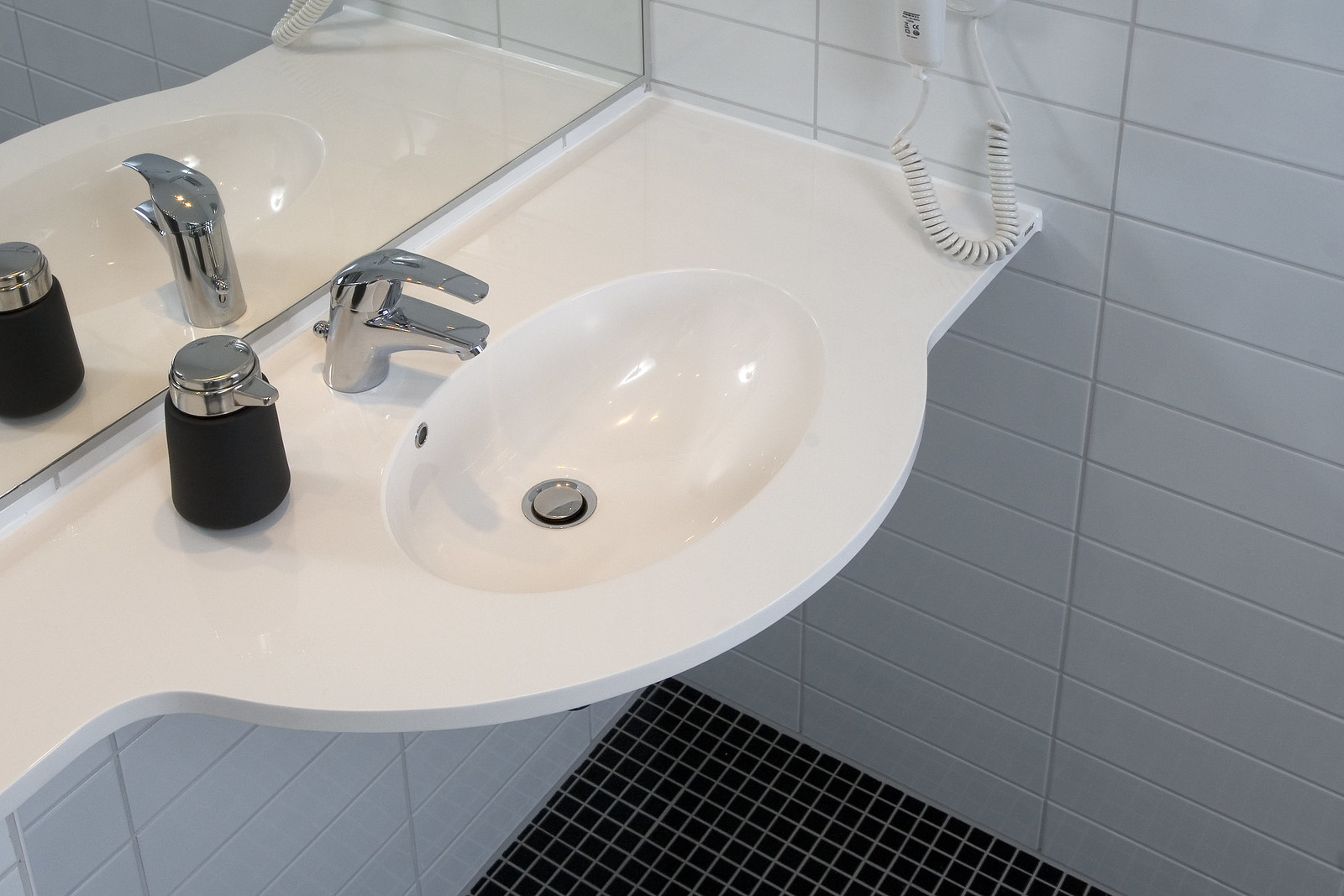A meticulously clean and modern hotel bathroom is showcased in this color photograph. The focal point is a pristine white sink that gently curves outward, paired with a sleek chrome faucet. The sink features a round silver drain at its base and is impeccably dry and spotless. To the left of the faucet, a cylindrical container with a silver top and black bottom stands out, possibly holding toiletries. On the right-hand side, a white cord trails from an object mounted on the tiled wall. The walls are adorned with white rectangular tiles grouted in light gray, adding a sophisticated touch to the scene. The floor contrasts elegantly with tiny black tiles bordered in light gray. A large mirror framed in chrome hangs above the sink, reflecting the minimalist and clean design of the space. This photograph, devoid of any people, seems perfectly suited for a hotel website, emphasizing the spotless and welcoming atmosphere of the bathroom.